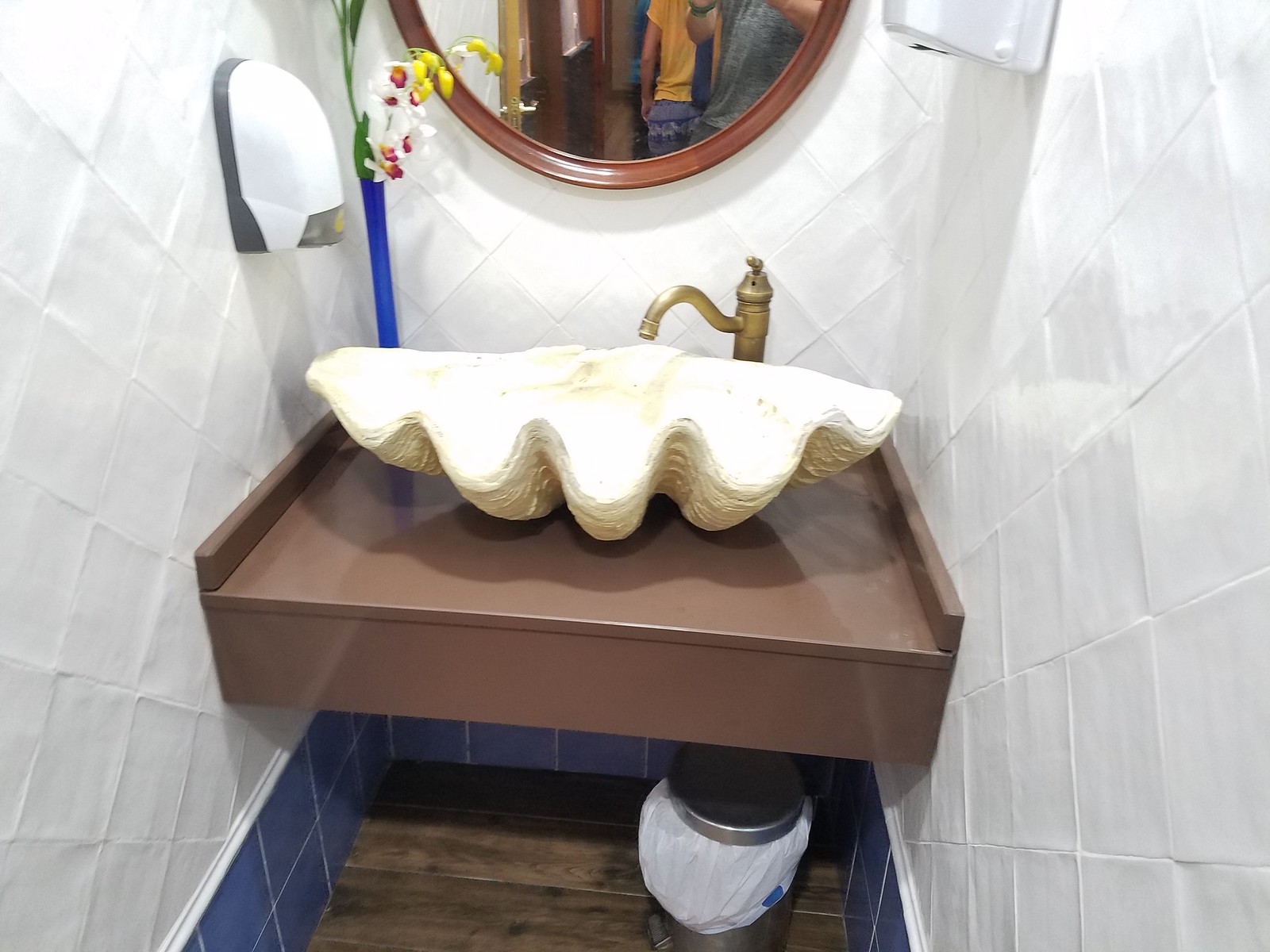The image depicts a narrow bathroom area, likely a commercial space, featuring a distinct seashell-shaped sink with a scalloped design. The sink is an off-white, slightly yellowish color, mounted on a brown painted countertop. A brass, ornate faucet with a single lever is installed on the upper right side of the sink. The bathroom walls are tiled with an off-white, diamond-shaped pattern, while a blue tile border runs along the bottom.

To the left of the sink, a commercial-style soap dispenser is attached to the wall, characterized by its white body and gray backing. Below the sink is a stainless steel, step-open trash can, partially lined with a white plastic bag. Ascending from the countertop is an oval mirror reflecting two individuals, likely the ones capturing the image. Adding a touch of decor, an artificial flower in a blue glass vase sits nearby. The overall setting is compact, measuring roughly three feet wide or about 30 inches, making efficient use of space to create a vanity area within the bathroom.